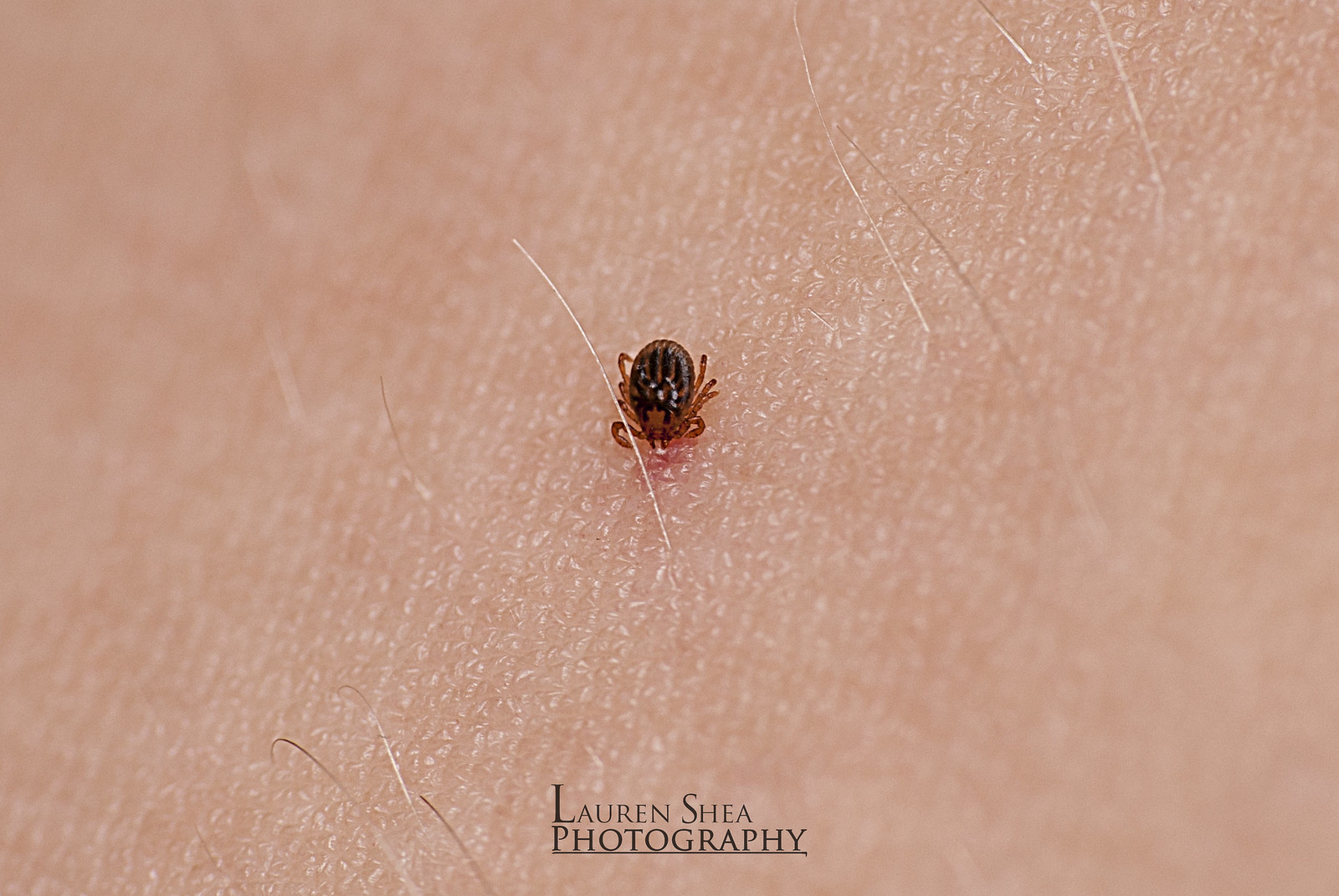This image, captured by Lauren Shea Photography, is an extreme close-up of a tick on human skin. The tick, which has a round, shiny back with dark brown stripes, is situated right in the center of the image, emphasizing its prominence against the textured surface of the skin. Its six small brown legs are visible, and the translucent nature of its body reveals darker internal structures. The skin around the tick is detailed, showing individual pores and a mix of sparse white and darker hairs. The edges of the photo blur slightly, drawing focus to the sharply detailed insect at the center, seemingly in the act of burrowing.